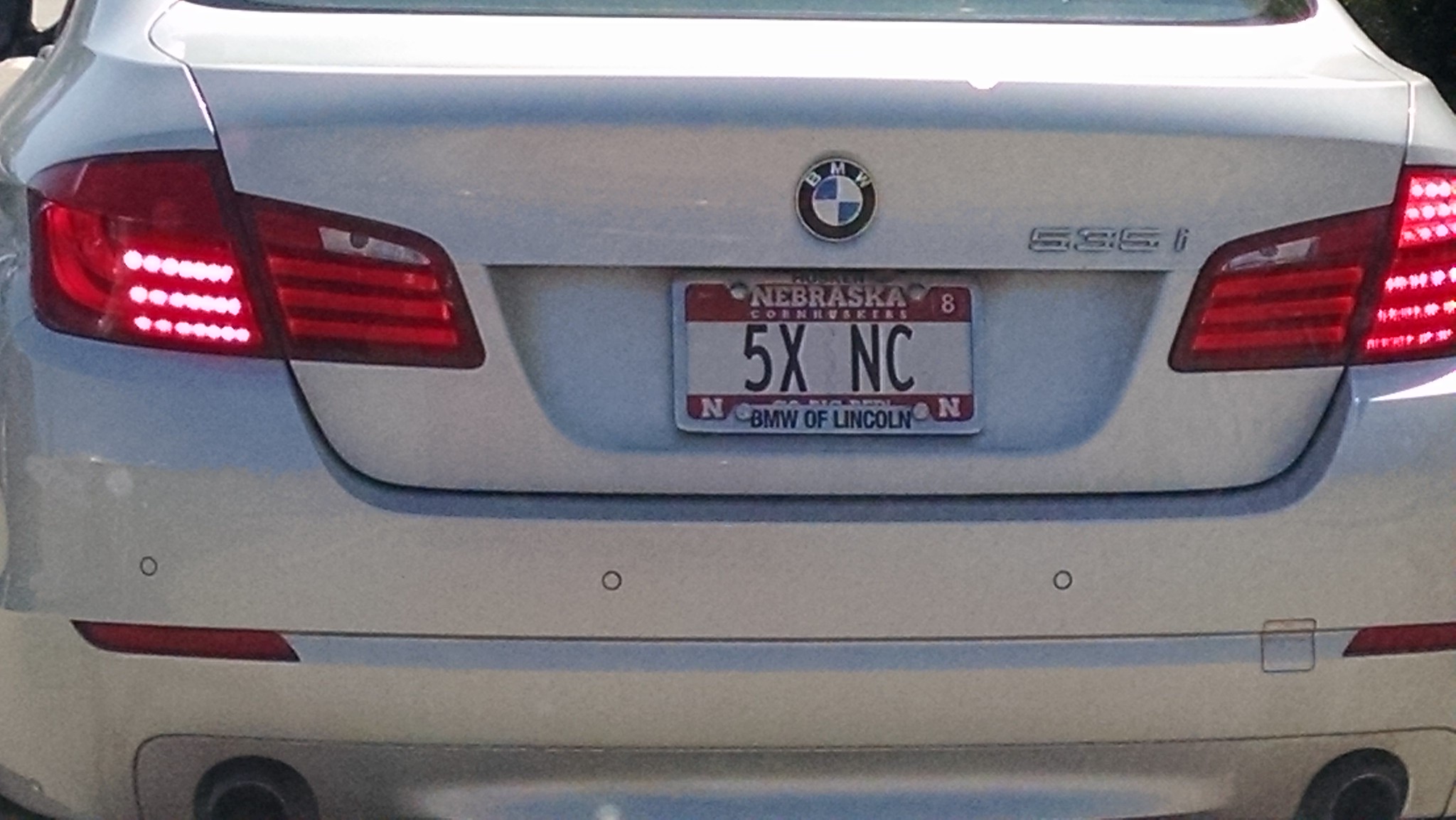This detailed photograph showcases the back of a white BMW sedan. The image centers on the vehicle's rear, capturing only the trunk and its immediate surroundings, excluding the wheels. The back lights are illuminated, emphasizing the car’s elegant design. Prominently featured in the middle is the classic BMW logo. 

The license plate, framed in silver, reads "5XNC" in bold black text on a white background, with "Nebraska Corn" inscribed above and below the alphanumeric sequence on a red background. The plate frame details "BMW of Lincoln," engraved at the bottom. The model designation, which appears to be either "535i" or "5351," is situated on the top right side, near the trunk handle. The surrounding space is dark, with a subtle white element on the left side of the image.